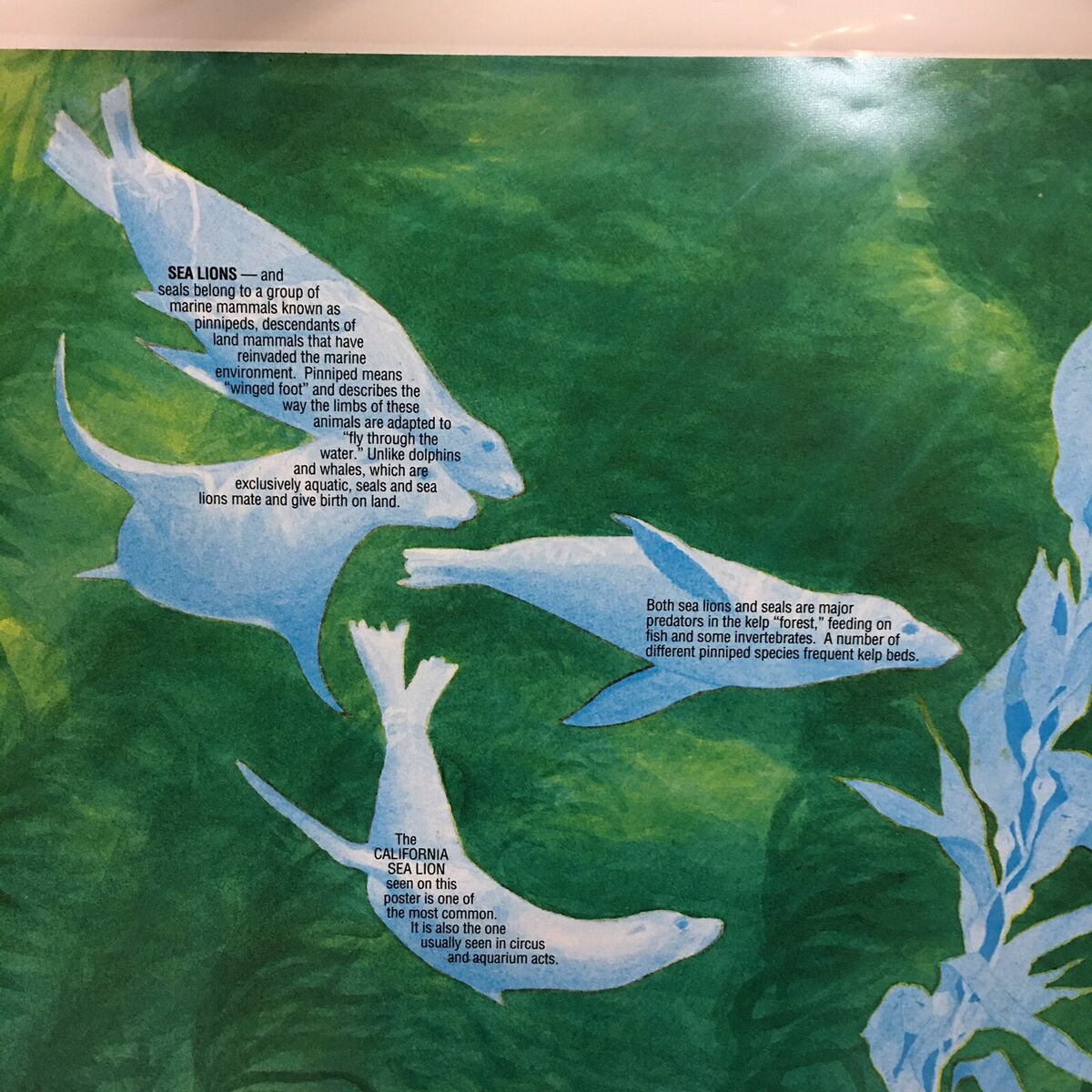This image is a detailed watercolor illustration, potentially a digital artwork, depicting an underwater scene teeming with marine life. The background is predominantly green, illustrating a vibrant kelp forest with various dark and light shades of green foliage that sway as if in currents. There is also a turquoise, viney, flower-like plant that adds to the rich underwater flora.

Amidst this lush kelp backdrop, four sea lions are depicted swimming gracefully. These sea lions are drawn in light blue and white hues, with some outlines and distinct features such as their flippers and tail flippers being discernible. Their small, dark blue eyes dot their faces, giving them a dynamic, lively look as they navigate through the kelp.

There is informative black text overlaying part of the artwork that reads: "Sea lions and seals belong to a group of marine mammals known as pinnipeds. Descendants of land mammals that have reinvaded the marine environment, pinniped means 'winged foot,' which describes the way the limbs of these animals are adapted to fly through the water. Unlike dolphins and whales, which are exclusively aquatic, seals and sea lions mate and give birth on land. Both sea lions and seals are major predators in the kelp forest, feeding on fish and some invertebrates. A number of different pinniped species frequent kelp beds. The California sea lion, seen in this illustration, is one of the most common and is often featured in circuses and aquariums."

Overall, this detailed illustration combines artistic skill with educational content, providing viewers with a visually appealing and informative depiction of sea lions in their natural underwater habitat.